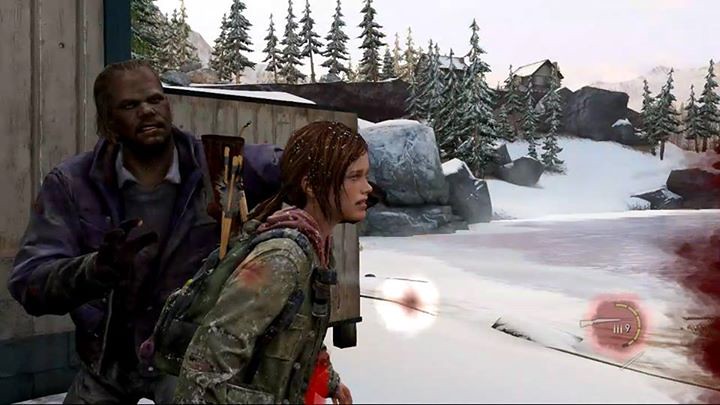In this highly realistic screenshot from what appears to be an apocalyptic-themed video game, a wintry landscape unfolds with snow-covered pine trees and mountains dotted with houses in the background. In the foreground, two characters are positioned near the lower left side, partially taking cover in front of a gray, vertically-lined building or storage unit. The image's leftmost character is an older, dark-skinned man dressed in a dark blue jacket, with a gruff or distressed expression. Beside him stands a young Caucasian girl with brown hair, clad in an army green jacket and carrying a backpack with arrows strapped to it. The contrast between the stark, snowy environment and the characters' detailed attire adds to the immersive atmosphere of the scene. In the lower right corner of the image, a red digital interface displays a drawing of a gun, three bullets, the number nine, and a semicircular bar, suggesting game-related information. The overall scene is set under a gray, bright daytime sky, further emphasizing the cold and desolate ambiance.